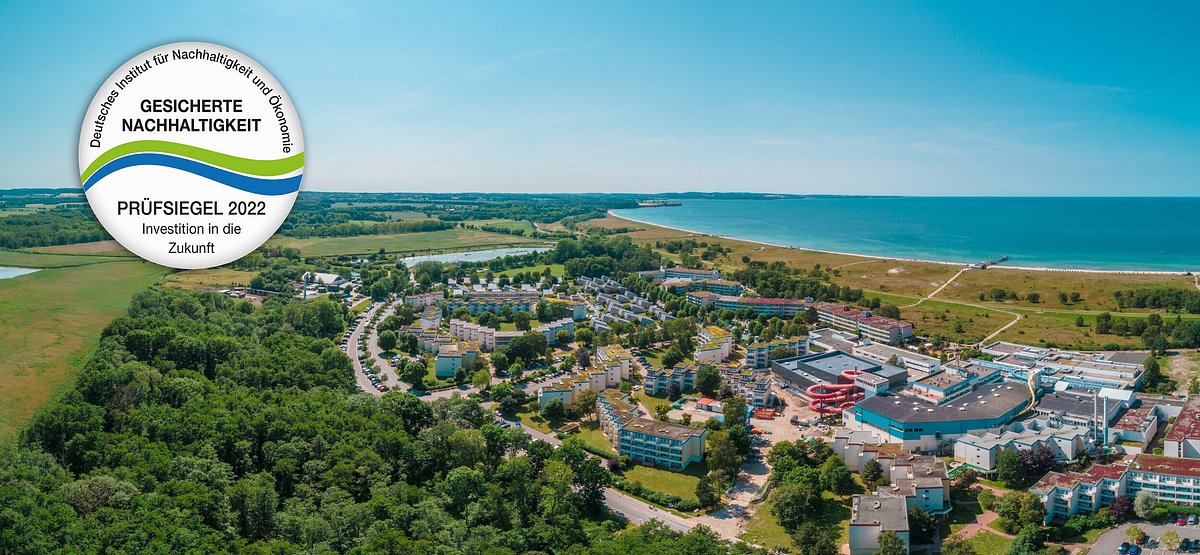This image, captured from above by a drone, shows a picturesque waterfront town. The view showcases numerous properties surrounded by roads, driveways, and parking lots. Sidewalks lead up to the waterfront, where the clear turquoise blue stretch of ocean meets the town. The landscape is enhanced by green grass and clusters of trees, providing a lush backdrop to the buildings.

Prominently featured at the top left corner of the image is a white circle containing German text and the year 2022. Inside this circle, two swooshes—one green and one blue—add a splash of color. The town below is a mix of vibrant blue buildings with red, brown, and charcoal gray rooftops. Cars are visible from the aerial view, navigating the town's layout. 

Further right in the image, the town transitions, showcasing a grand building with large, red tubular structures that seem to be waterslides. Adjacent to this is a sizable blue and white building. Beyond the town, the brilliant turquoise ocean seamlessly blends into the equally vibrant sky, creating a serene and inviting atmosphere.